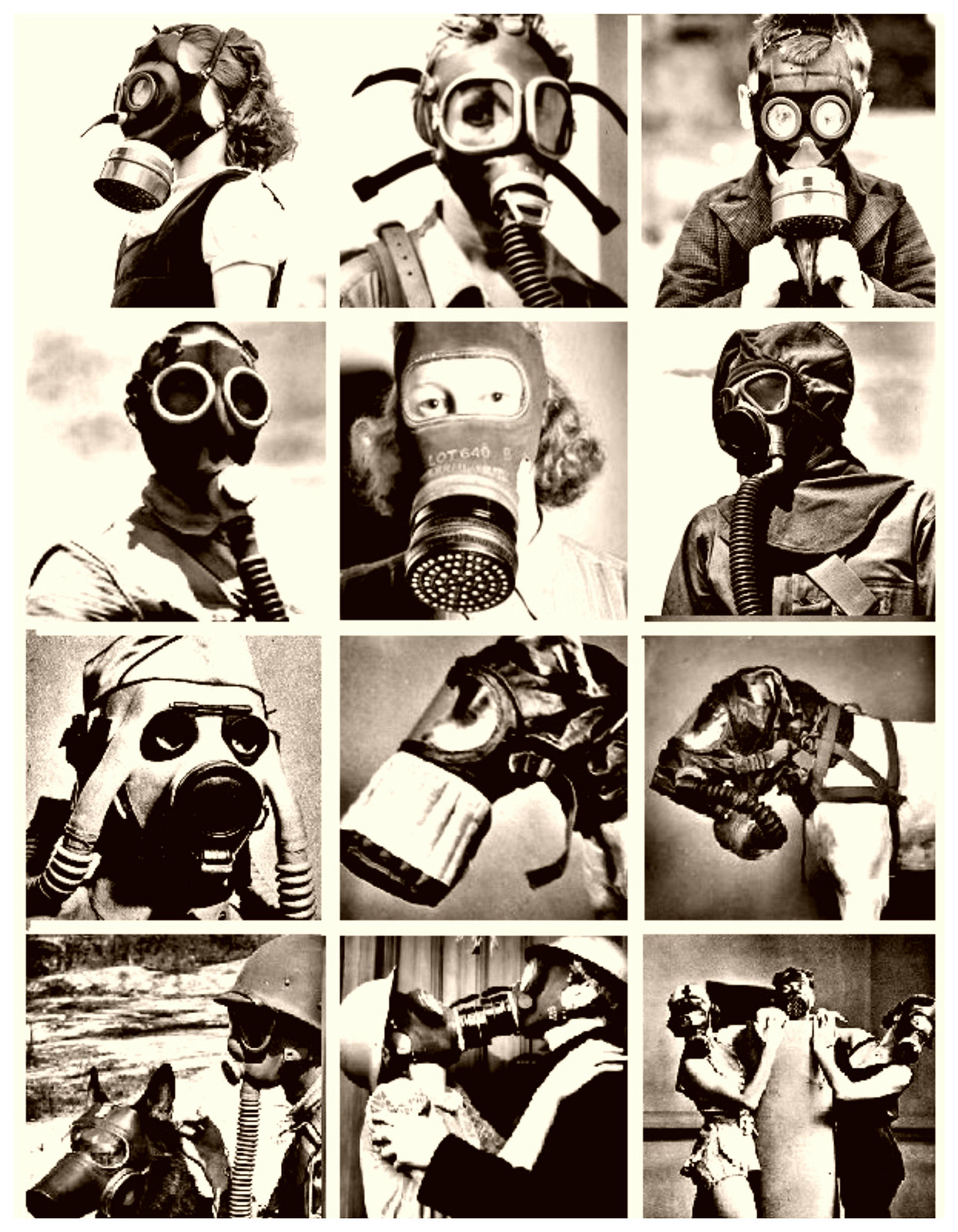A striking, black-and-white montage consisting of twelve square photographs organized in four rows of three. Each image presents a person or animal donning a gas mask, featuring a variety of designs that include filters, circular cylinders, and rubber tubes extending from the masks' mouths. Amongst the individuals, there are men, women, and children, each captured from various angles—profiles and direct eye contact with the camera.

The top row features a woman's profile, another woman facing the camera, and a boy gazing directly at the viewer. In the second row, several men face the camera, their expressions obscured by their masks. The third row is anchored by two dogs wearing different styles of gas masks, both in profile, alongside a man also in a gas mask. On the bottom row, the far left photo shows a man in an army helmet standing next to a dog, both equipped with rubber-tubed masks. The center image is a poignant scene of a man and woman kissing, their gas masks pressed together as they embrace. To the right, three figures—two women and a man—pose in an elaborate setup that appears almost theatrical, wrapped in fabric and evoking a sense of drama.

The diverse gas mask designs vary in complexity, some with darkened eye lenses and others that offer a clear view of the wearers' eyes, contributing to the hauntingly surreal and thought-provoking nature of the composition. Among these individuals, there is a conspicuous inclusion of animals—dogs in the central panel and what appears to be a horse or another dog next to a helmeted soldier—further emphasizing the pervasive, unsettling atmosphere of the era this series seems to depict, likely around the 1940s or 1950s.